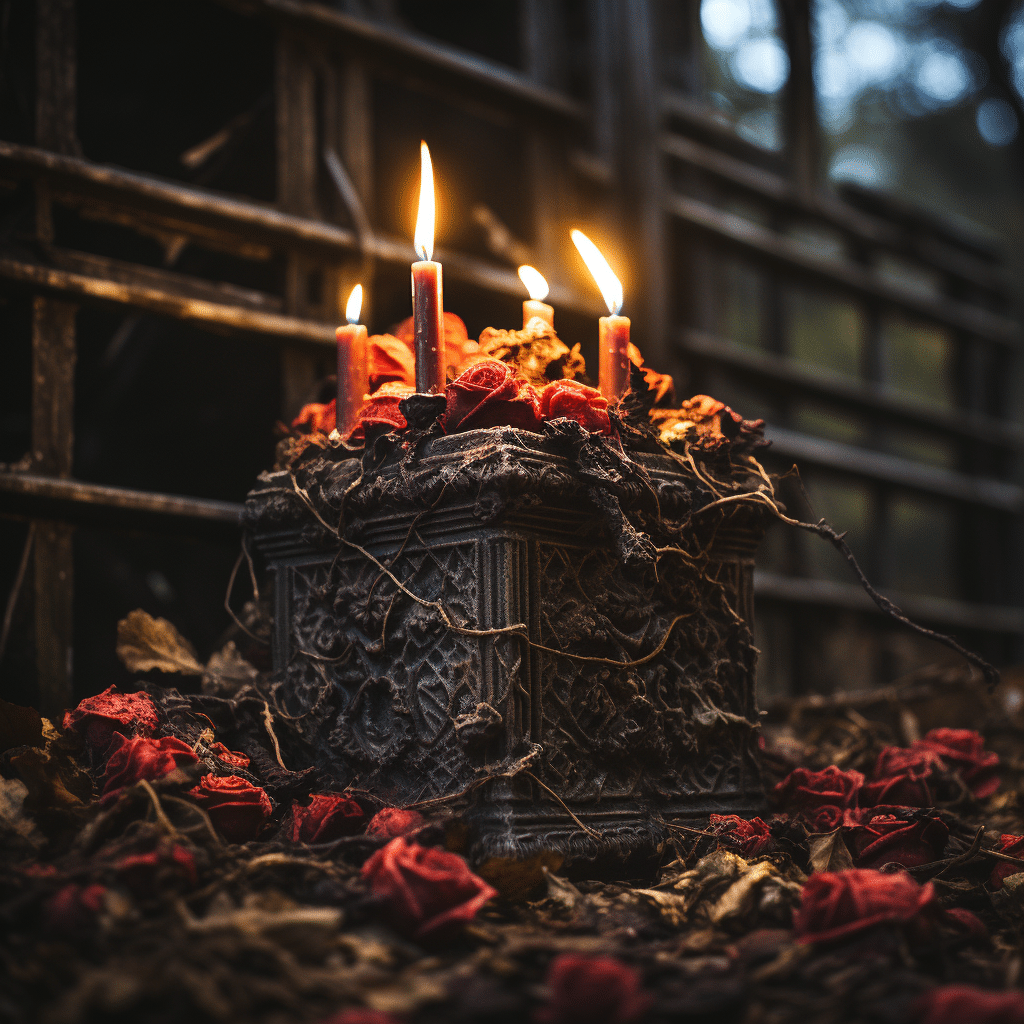The image showcases the interior of a dilapidated, gothic-style church or similar structure. At the center of the scene is an ornately carved box, which might be made of wood or stone. The carvings are highly elaborate, potentially featuring intricate designs or faces that are difficult to discern due to the image's blurriness. This box, resembling a sacred or ceremonial item, is adorned with four lit red candles, one at each corner, casting a somber glow in the darkened space.

Surrounding the box and spilling over its lid are numerous dried red roses, rose petals, and scattered plant matter, making the scene feel like a memorial or altar. Twining around the box are dried vines, adding to the sense of decay and timelessness. The setting is filled with a dark, gothic ambiance, with dead branches and lifeless flowers scattered on the floor, which all contribute to the overall atmosphere of mourning or remembrance.